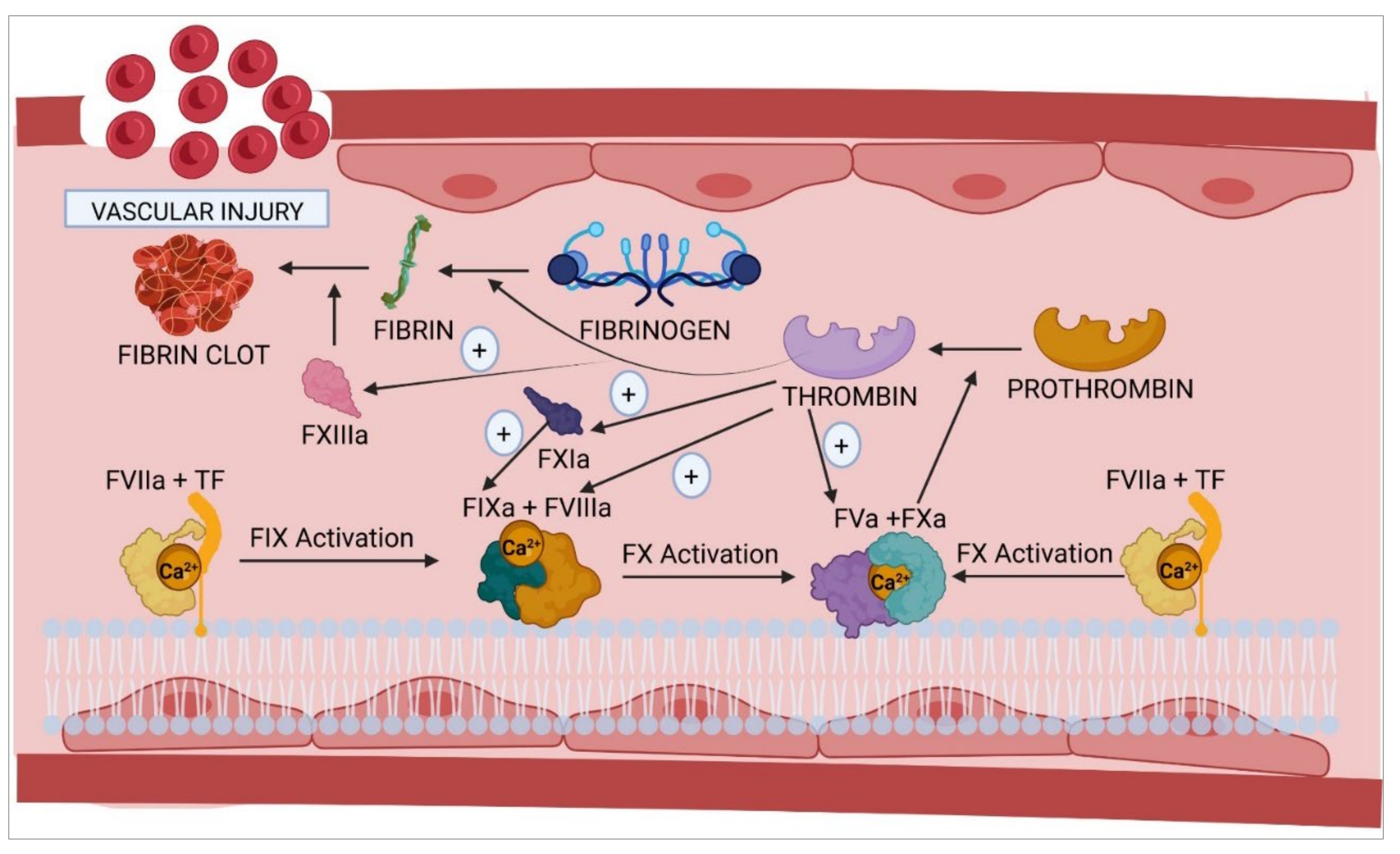The image depicts a detailed, cartoonish diagram of a biological pathway, likely the interior of a vein or a part of the cardiovascular system, emphasizing a vascular injury and ensuing clot formation processes. The diagram is rectangular, about five inches wide and three to four inches high, with a thin black border enclosing a white outline.

At the top and bottom of the image, there are dark reddish-pink horizontal lines, inside of which sit medium pink, rounded, inverted triangular shapes with darker pink tips. These lines frame a light pink background. Within this framework, cells and various components related to blood clotting and vascular injury are illustrated using different colors for clarity.

In the upper left corner, blood vessels are illustrated, with a small gray-background text box labeled "vascular injury" underneath. The diagram showcases numerous interconnected parts and labels, depicting components like fibrinogen, fibrin, thrombin, FIX activation complexes, calcium deposits, and other cell parts involved in clotting.

Numerous arrows and plus signs connect these components, illustrating the activation processes and interactions. Key visual elements include a fibrin clot labeled at the top, and differently colored blobs (yellow, green, purple, bluish-green) scattered throughout, each indicating specific biochemical elements like FV11A plus TF leading to FIX and SX activation. The sequence culminates back at the fibrin clot, depicting the dynamic and multifaceted response to a vascular injury. This comprehensive diagram effectively communicates the complex biological pathways involved in vascular injury and clot formation.